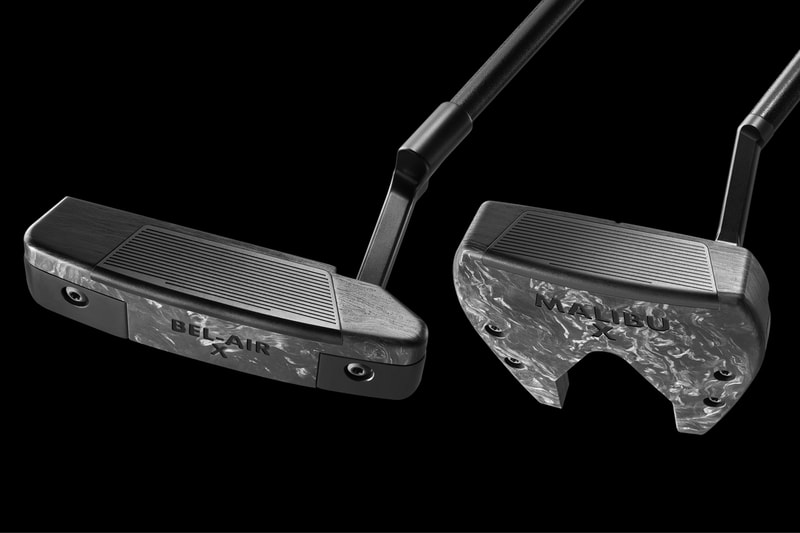The image features a meticulously captured, professional-looking photograph set against a stark black background. In the center are two distinct objects, initially resembling golf putters due to their elongated shafts and angled heads, but upon closer inspection, are revealed to be car pedals – a brake and a gas pedal. The brake pedal is labeled "Bel Air X" and the gas pedal is marked "Malibu X", both in white text. These pedals are rendered in monochromatic tones of black, gray, and silver. The foot pedals attach to a connecting bar, mimicking the profile and shape of golf clubs. The photograph, devoid of any additional context or surrounding elements, solely focuses on these pedals, highlighting their mechanical design and metal finish.